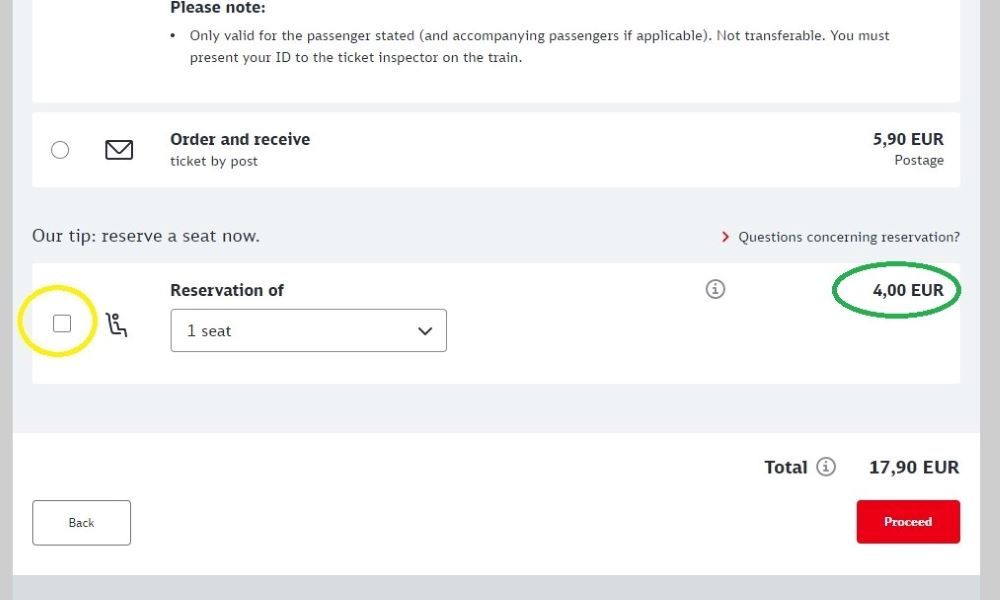The image depicts an online reservation process for a train ticket. At the top left, there is a notice with the bold text "Please Note:" followed by instructions in regular font: "The following is only valid for the passenger stated, and accompanying passengers if applicable. Not transferable. You must present your ID to the ticket inspector on the train."

Below the notice, there is an icon resembling an envelope, and to its right, bold text reading "Order and Receive." Beneath this, in standard font, it states "Ticket by Post." Further to the right, there is a price listed as "5.90 EUR" accompanied by the label "Postage."

Below this section, a tip is provided: "Our tip: reserve a seat now." Adjacent to this tip is a yellow-circled checkbox next to an icon of a person reclining in a chair. To the right, it states "Reservation of 1 seat," with a descending arrow indicating a dropdown menu. The cost for this seat reservation is listed as "4.00 EUR," encircled in green.

At the bottom of the form, the total cost is displayed as "17.90 EUR." Finally, at the very bottom, there is a prominent red button labeled "Proceed."